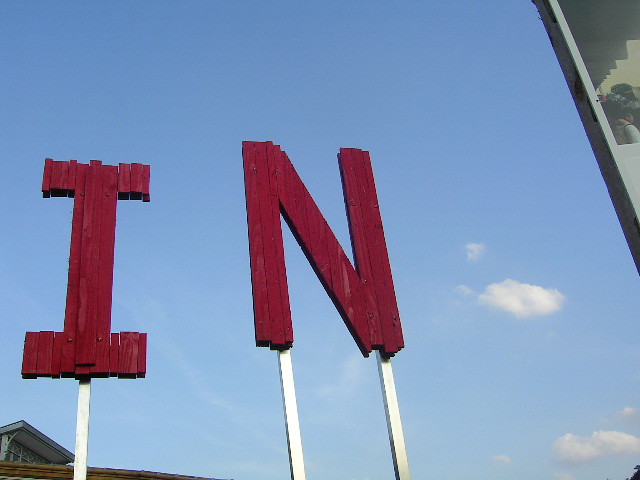This photograph captures the last two letters of a sign, featuring a large red capital "I" and a capital "N" made of wood and painted in a maroon-red color. The sign is attached to white poles and set against a bright blue sky sprinkled with a few small, puffy white clouds. The letters "I" and "N" are positioned slightly off-center towards the left side of the image. At the bottom left corner, you can see the very top of a brown flat-roofed building, which the sign seems to be mounted on. On the right side of the image, there is a glimpse of a gray structure that could be part of another building or a billboard, featuring a face that seems to be wearing a helmet. Additionally, a tiny smidge of a tree is visible in the lower right corner, hinting at more elements beyond the frame. The overall scene hints at a larger environment, possibly a stadium or racing track, but the focus remains on the bold, red letters against the sky.